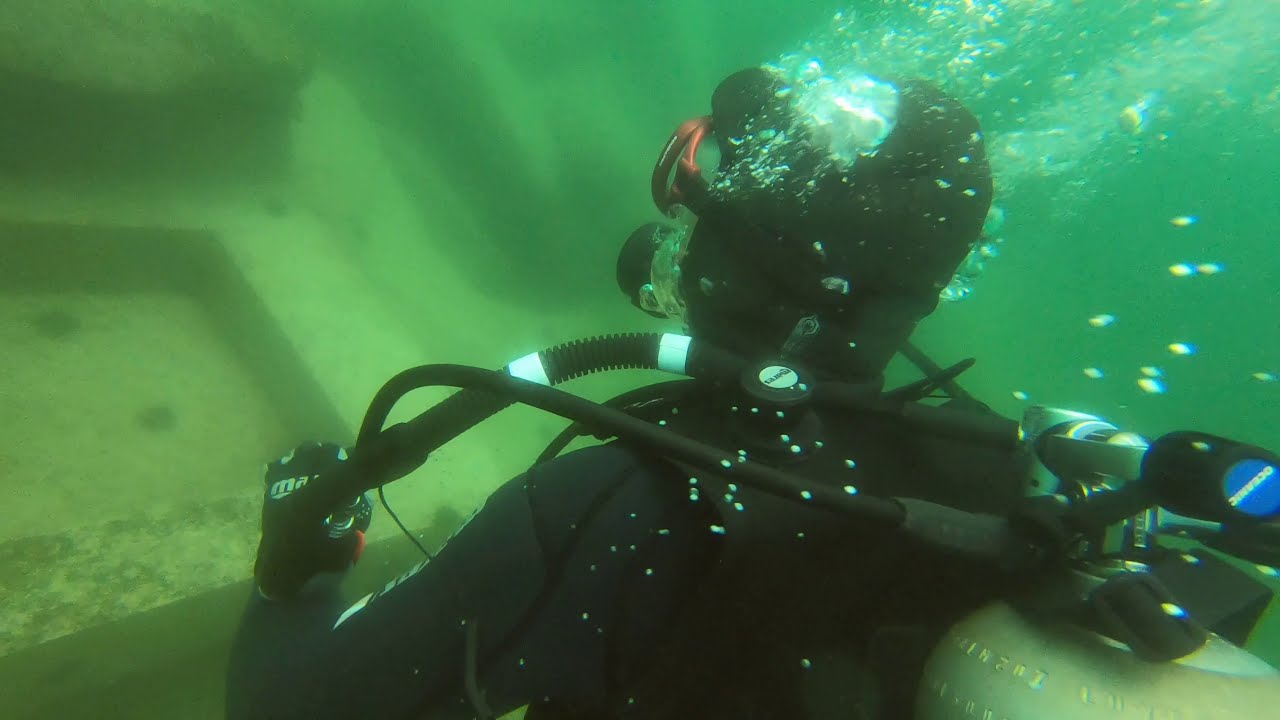The image captures an underwater scene dominated by a scuba diver in a black wetsuit and red-rimmed goggles, positioned centrally with only their top half and head visible. The diver is exhaling bubbles, which float around their head, and wearing gloves with white wording. They carry a yellow and tan air tank on their back, connected by black pipes to the front of their suit. The water around them has a murky green-gray hue, with variations in color: a bluish-green on the right and a yellowish-green on the left. The left side of the image also reveals various concrete or man-made shapes on the bottom, suggesting the presence of an underwater structure or ruin. No marine animals are visible in the scene.